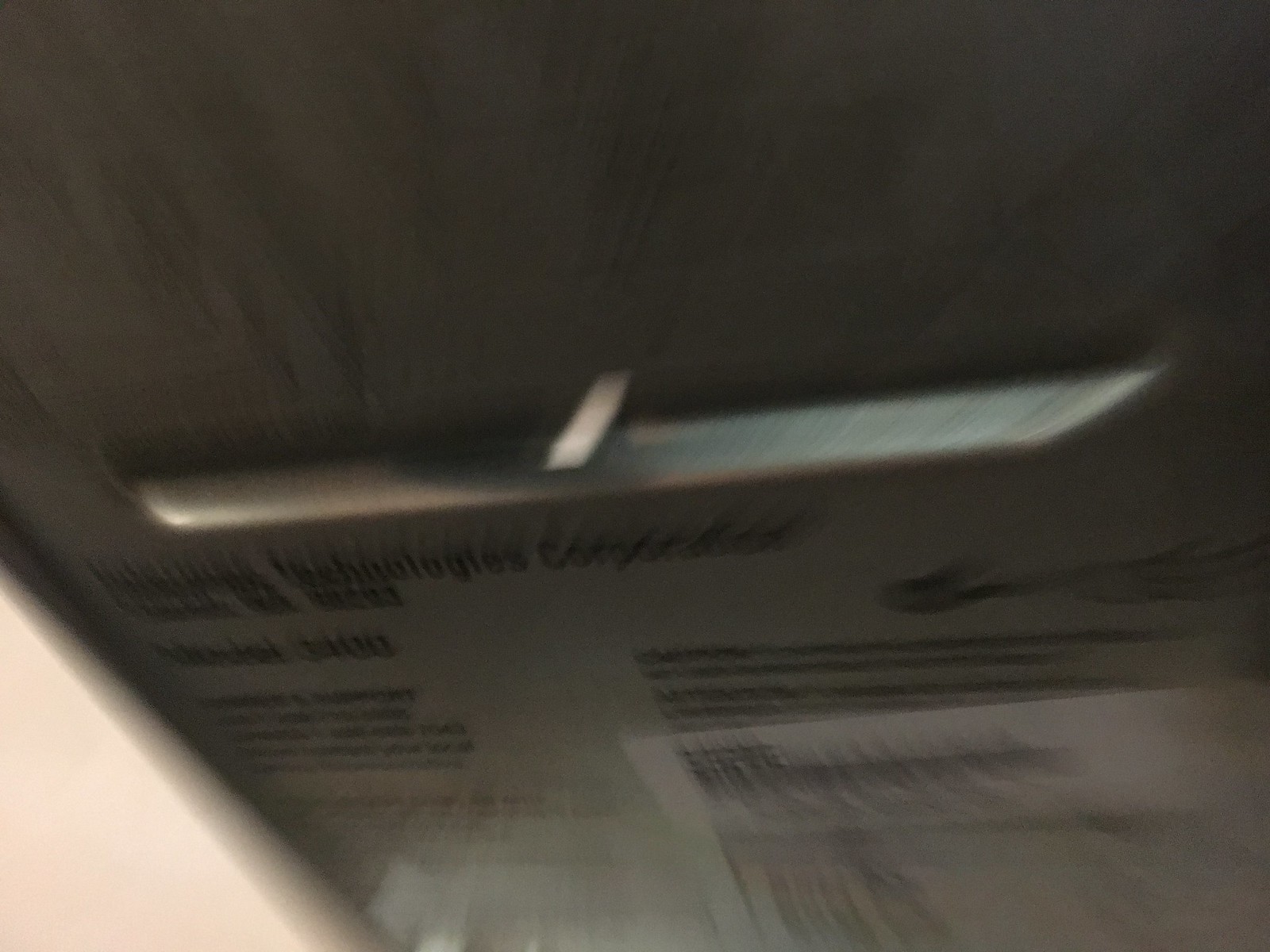A highly blurred photograph captures what appears to be a label affixed to an object, possibly related to medication or a prescription. The photo, taken with significant motion blur, suggests the camera was moved rapidly upward and backward during the shot. This results in elongated, vertically-stretched text that is difficult to decipher. While the specific words remain unreadable, the label itself is distinguished by its white color contrasting against a darker background. The details on the label could potentially be directions or contents, although the exact purpose remains unclear due to the image's blurriness.